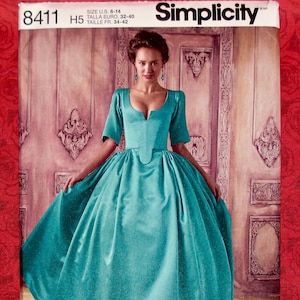The image is an advertisement set against a red background, featuring a red thin border on both the left and right sides, as well as at the top. The prominent black bold text reads "Simplicity" with a serial number "8411" and information indicating US sizes 6 to 14. The main section displays a photograph of a young lady modeling a satin teal ball gown. The dress is full-length with a flaring skirt and half-length sleeves that reach the elbows. It has a fitted bodice with a V-neckline and a low front cleavage, giving it an elegant and somewhat old-fashioned princess style. 

The model has brown hair styled into a bun on top of her head, contributing to a vintage look. Her features include a beige complexion, soft eyebrows, small eyes, a small nose, and small pink lips. She is set against a background with a tan and pinkish-tan center adorned with patterns that resemble a man's face with a beard. The model's pose highlights the expansive flare of the gown, holding the fabric out to each side to emphasize its voluminous design.